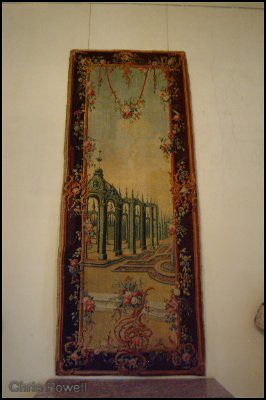The image showcases a piece of artwork prominently displayed against a white wall. The artwork is an old, intricate carpet characterized by a brown border and a detailed black frame within. The carpet features a rich tapestry of designs including green leaves, flowers, and architectural elements reminiscent of a castle or temple. The central image within the carpet depicts a scene with a silver-colored castle, a park, and a bright blue sky. Pink and red flowers add vibrant touches to the mostly warm, earthy palette that includes hues of brown, blue, red, and green. Additionally, the carpet artwork is suspended by two lines from the ceiling, giving it an elevated presentation. Below the artwork sits a reddish granite-like table, adding a solid base to the display. The name "Chris Powell" is inscribed in white in the bottom left corner of the carpet. The overall setting exudes an old-school charm with a slightly dull yet warm ambiance.